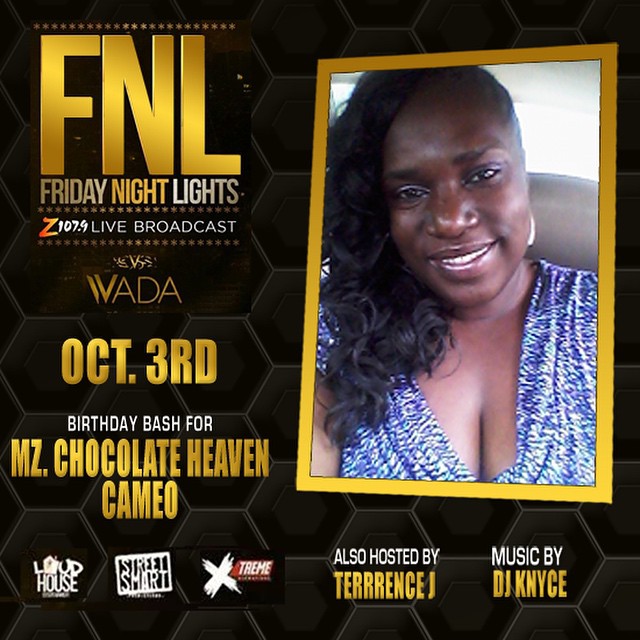The image features a detailed advertisement for an event. At the top, large gold text reads "FNL," followed by "Friday Night Lights" and "Z107.9 Live Broadcast" in white text. Further down in gold lettering, the event details include "October 3rd," and "Birthday Bash for MZ Chocolate Heaven Cameo." Surrounding the text, a honeycomb-patterned brown background adds texture to the design. The advertisement also features logos for sponsors at the bottom: Loud House, Street Smart, and Xtreme. On the right side of the flyer is a prominent image of a black woman with long, curly hair, brushed to one side. She is wearing a shiny blue blouse and appears to be sitting in a car, with a seat rest visible behind her and a bright, glary background through a window. Below her image, text in white indicates the event will be hosted by Terrence J. with music by DJ Kints.